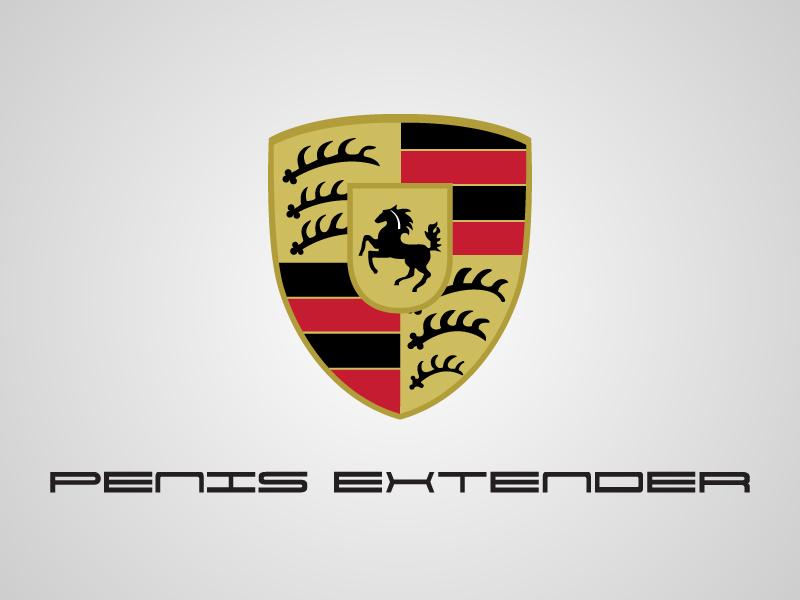The image depicts a professionally-designed emblem resembling a traditional British shield, predominantly featuring a central black horse with a white streak on its head. The shield's intricate design includes gold outlines and a combination of black, white, mustard, and red colors. The emblem is adorned with red and black stripes in the lower left and upper right corners, and jagged sword-like shapes in the upper left and lower right corners. Below the emblem, the text "PENIS EXTENDER" is displayed in capital letters in black, using a font reminiscent of the Blade Runner style. The entire logo rests on a white background, showcasing a sophisticated and detailed composition.